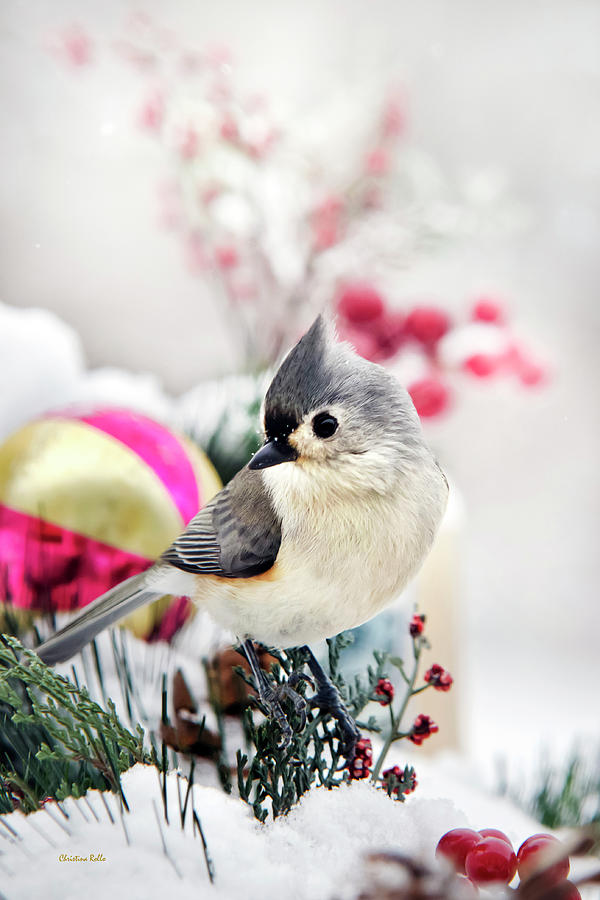The image features a highly detailed and realistic depiction of a small bird perched amid a winter scene. The bird, which has light cream feathers on its belly and gray feathers on its head, wings, and tail, is poised as if about to take flight. It also has a bit of orange under its wings, adding to its life-like appearance. Its small black eyes and beak are distinct against its delicate features. The bird gazes over its shoulder towards the bottom right, with its body oriented towards the right but its head turned to the left. It stands with its tiny black feet on a surface covered in ice and lightly dusted snow.

Surrounding the bird, there is an array of greenery, including blades of grass, leaves, and little pine needles, interspersed with stems bearing red and dried berries. Some flowers in red and pink hues add a pop of color to the otherwise wintry landscape. In the background, a gold and pink striped ornament peeks through the foliage, adding a festive element to the scene. The entire setting is winter-themed, with twigs and sticks adorning more red berries, wrapping up the detailed and vibrant tableau. In the bottom left corner, an artist or photographer has signed the image, emphasizing its crafted nature.